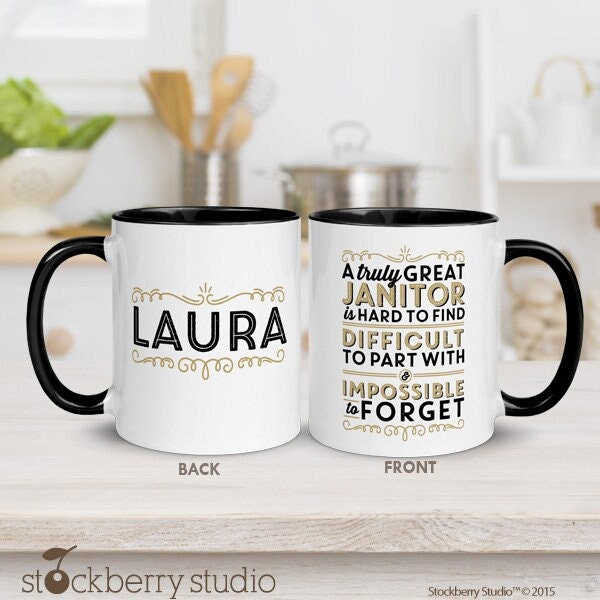In a cozy, bright kitchen setting, two white ceramic coffee mugs with black interiors and handles are prominently displayed side by side on a light gray wooden countertop. The mug on the left, labeled "Back" in gray letters below it, features the name "Laura" in large black text surrounded by intricate golden vine designs at the top and bottom. The mug on the right, labeled "Front" in gray letters below it, bears a heartfelt message: "A truly great janitor is hard to find, difficult to part with, impossible to forget." The text is artistically varied in black and tan colors, with decorative horizontal lines enhancing its presentation. Behind the mugs, the blurry background reveals a kitchen scene with a white wall, wooden utensils in a holder, a stainless steel pot, a bowl of green lettuce, and other kitchen essentials. At the bottom of the image, "Stockberry Studio" is inscribed in gray text along with a distinct cherry logo in the letter 'O' and '2015' marking the date. The scene captures a homely atmosphere, emphasizing the sentimental value and personalized nature of the coffee mugs.